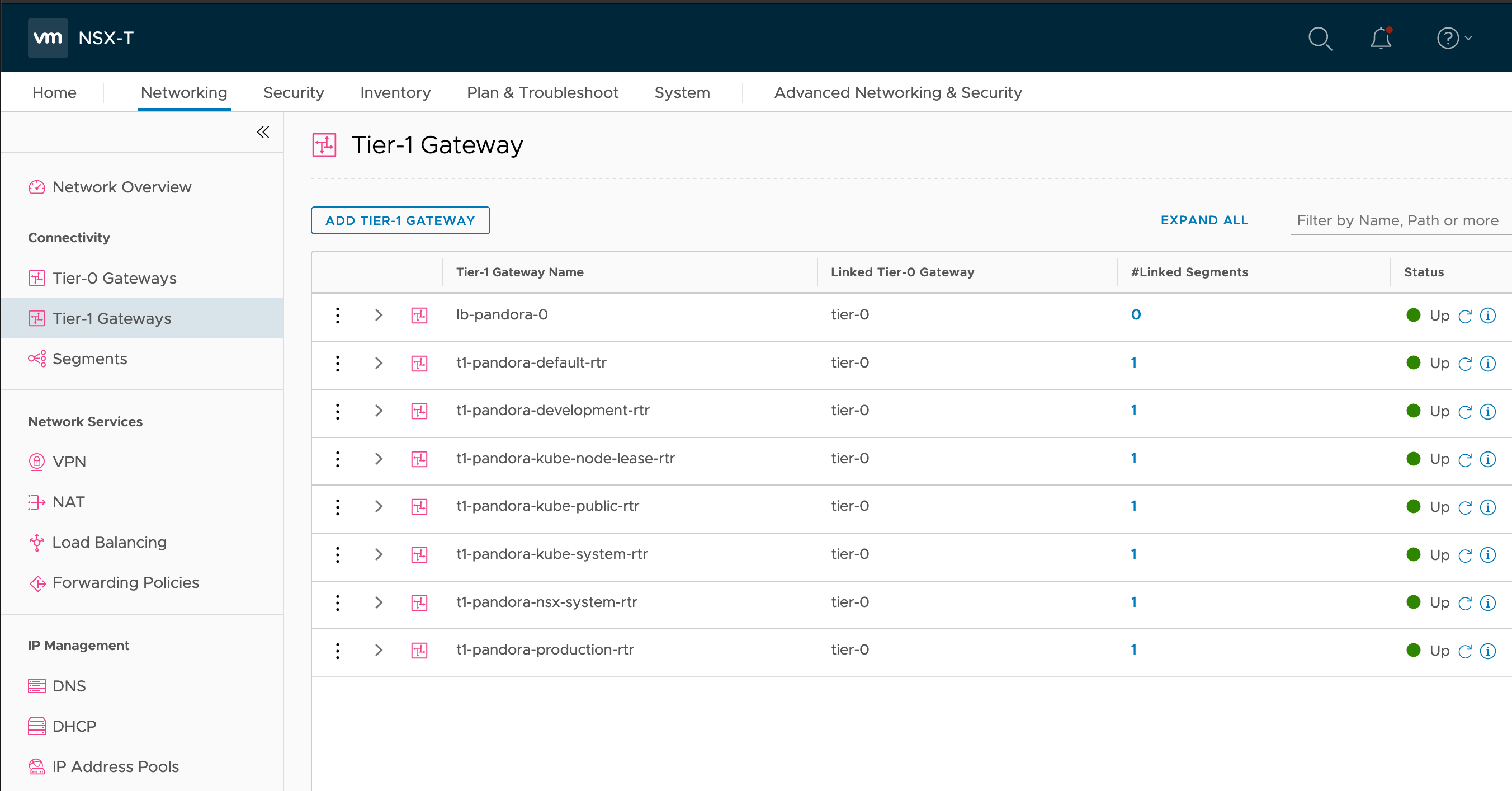A detailed descriptive caption for the image could be:

"The screenshot captures a detailed web page interface of VM NXT, prominently featuring a top banner with options for a search engine, notifications, and question assistance. Below the banner, there is a navigation bar with several tabs including Home, Networking, Security, Inventory, Plan and Troubleshoot, System, Advanced Networking, and Security. The current tab selected is 'Networking'. On the left sidebar, there are various sub-categories such as Network Overview, Connectivity, Tier 0 Gateways, Tier 1 Gateways, Segments, and a section for Network Services which includes VPN, NAT, Load Balancing, Forward Policies, and IP Management services like DNS, DHCP, and IP Address Pools. The interface is currently displaying the 'Tier 1 Gateways' section. In this section, users have options to add various configurations to the Tier 1 Gateway, with detailed descriptions for each option, that might be complex for the layperson. This includes fields for Gateway Name, Linked Gateways, Linked Segments, and Status. All listed gateways are operational as indicated by their statuses, with 'Pandora' being the primary gateway name repeated throughout the list."